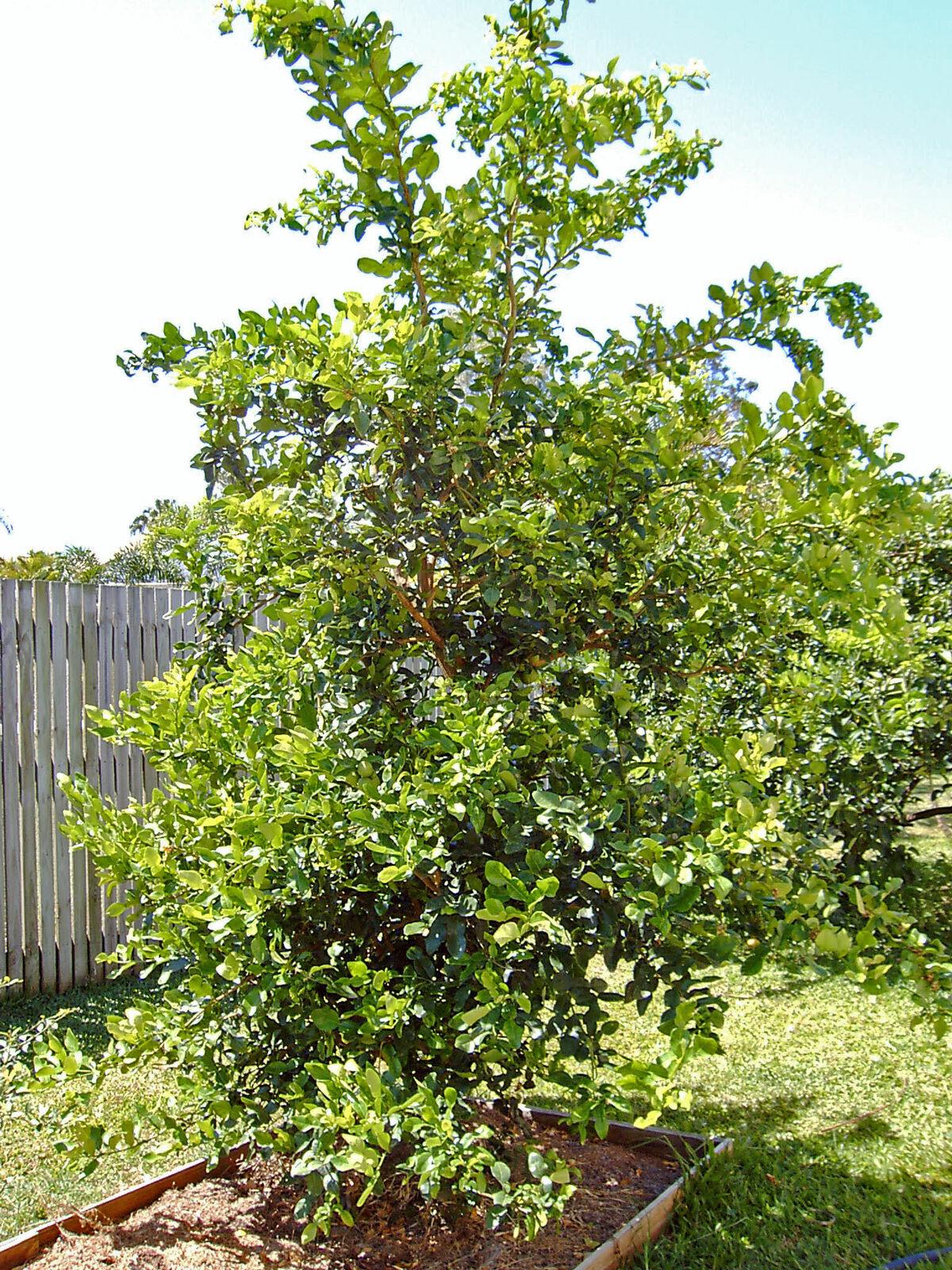The image captures a fruit-bearing juvenile tree, likely a lemon tree, standing in the middle of a backyard during a bright, sunny day. The tree, approximately seven to eight feet tall, has thick branches adorned with broad, dense foliage that obscures the trunk. Within its greenery, a few yellow fruits can be spotted. The tree is planted in a raised rectangular bed, framed by two-by-fours and filled with light brown mulch. Surrounding this bed is a neatly mowed lawn, extending towards a diagonally positioned lot. In the background, a four to five-foot-tall wooden slat fence runs along the left side, and the bright sky above gives the image an overexposed look, casting shadows underneath the tree. The raised bed continues beyond the tree, suggesting the cultivation of additional plants, not visible in the image.